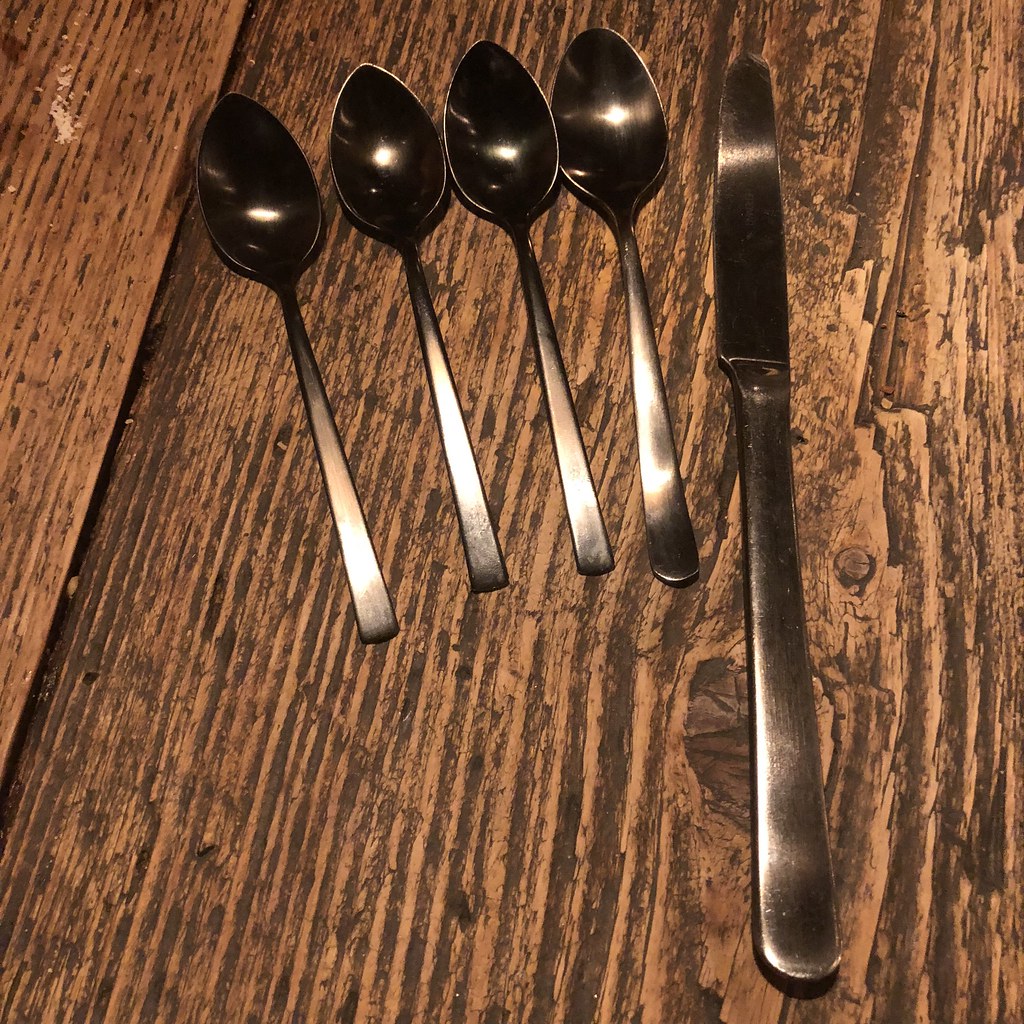This color photograph captures a rustic setting featuring five pieces of silverware laid meticulously on a weathered, medium-brown wooden table with visible grain and dark brown streaks. At the center of attention are four shiny, silver spoons positioned side by side in a straight line near the top of the image. Three of the spoons boast long, slender handles that terminate in sharp, rectangular edges, while the fourth spoon, closest to the knife, has a slightly bulkier build with a rounded handle, suggesting it might belong to a different set. Adjacent to these spoons, and extending from the bottom of the image upwards, is a lengthy butter knife, notable for its disproportionately long handle compared to its short, dull blade. Both the knife and the rounded spoon handle display light reflections, accentuating their shiny surface, and minor wear such as scratches. The table beneath the silverware has uneven, rough-hewn boards with minor scarring and crumbs in the upper left corner, hinting at a rustic, well-used kitchen environment. The lighting in the photo highlights the utensils' reflective surfaces and gives the table hints of pink tones, adding to the photograph's overall artisanal quality.